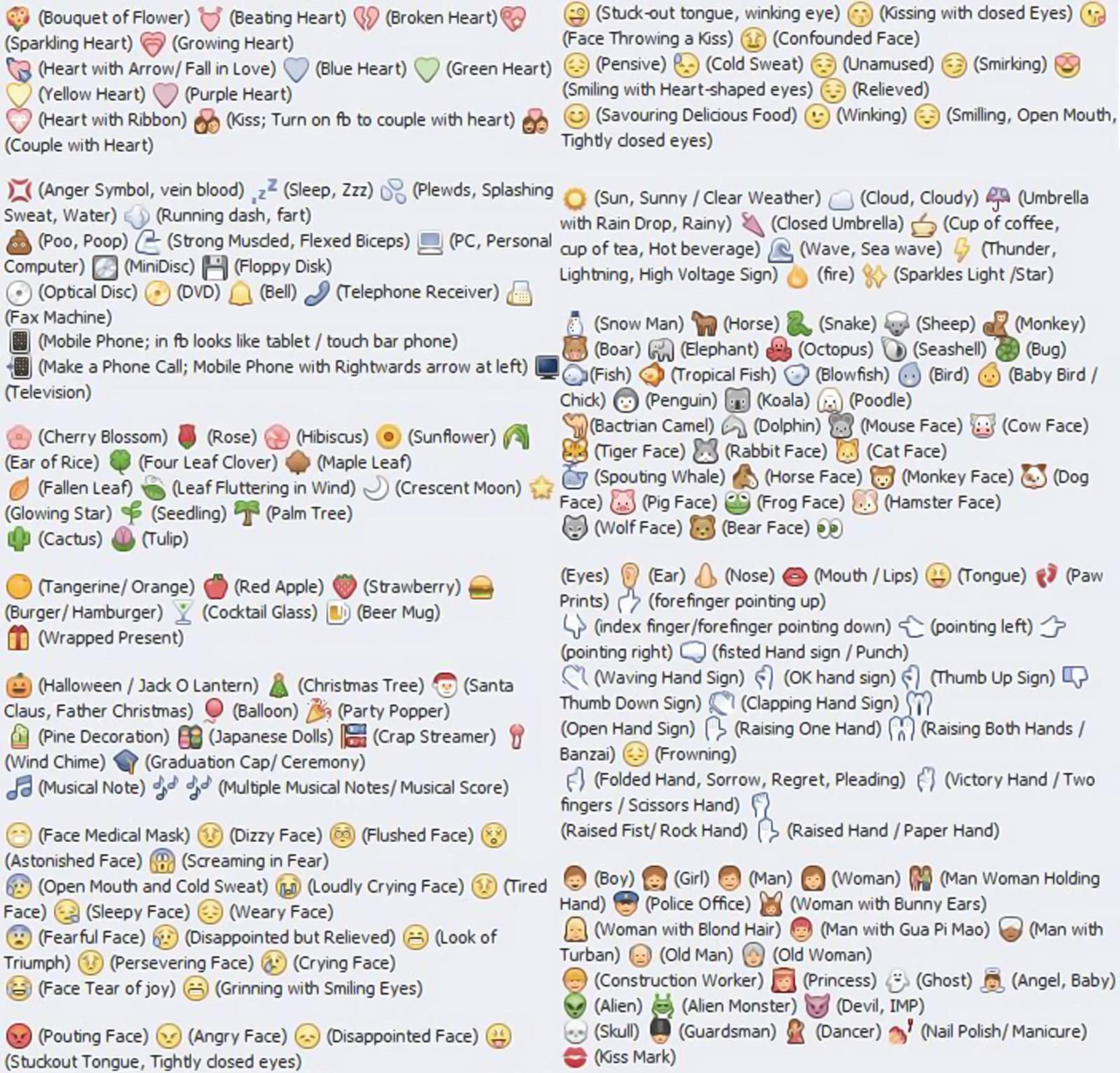The image presents an extensive collection of social media emojis and icons arrayed against a light blue background. The layout resembles a giant list or a webpage, divided into two columns filled with a multitude of colorful emojis. Each emoji is accompanied by its corresponding description in black text. Starting from the upper left corner, various emojis like the bouquet of flowers, which is labeled "bouquet of flower," and the beating heart, labeled "beating heart," are displayed. This pattern continues with the broken heart, fruit, vegetables, smiley faces, and more. A comprehensive range of emojis includes smiley faces, sun, clouds, animals like horses, snakes, and monkeys, as well as body parts such as ears, noses, eyes, and hands making different gestures. There are emojis of objects like a personal computer, floppy disk, mobile phone, and television. Nature and event-themed emojis like cherry blossoms, Christmas trees, and Santa Claus are also present. The image is vibrant, featuring a palette of colors: red, orange, yellow, green, gray, black, light blue, and white, densely packed, with very few blank spaces, creating an exhaustive visual list of emojis.